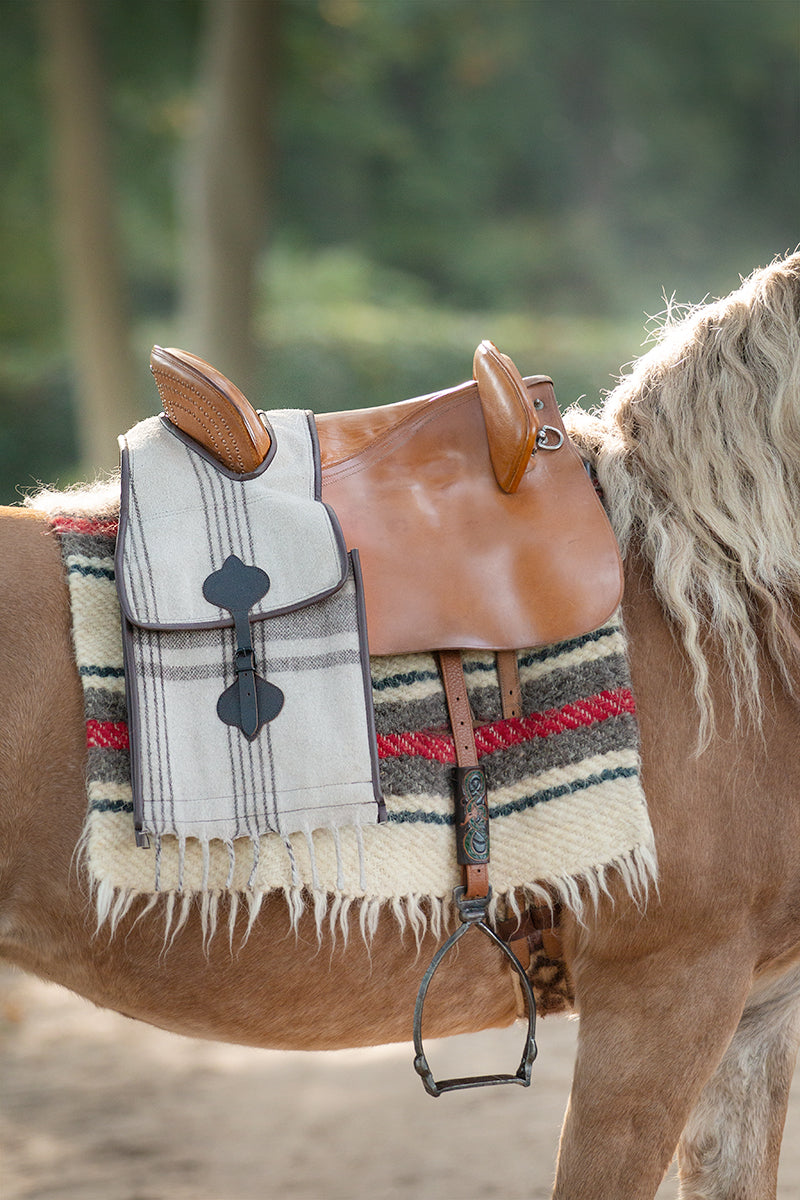This vertical, rectangular image captures a side view of a light brown horse with a yellow-white, scraggly mane that appears unbrushed. The focus is primarily on the horse's midsection, showing its front legs and part of its back but omitting its head and tail. The horse, standing on light beige dirt, is outfitted with a saddle and a blanket. The blanket, which appears handmade, is cream-colored with thin gray stripes and a prominent thick gray stripe bordered by red. The caramel-colored leather saddle, an English type, is small and sleek, featuring bars in the front but lacking a horn, with stirrups hanging down its sides. A white and gray saddle bag hangs over the back of the saddle. In the blurry background, green trees, bushes, and two brown tree trunks are visible.